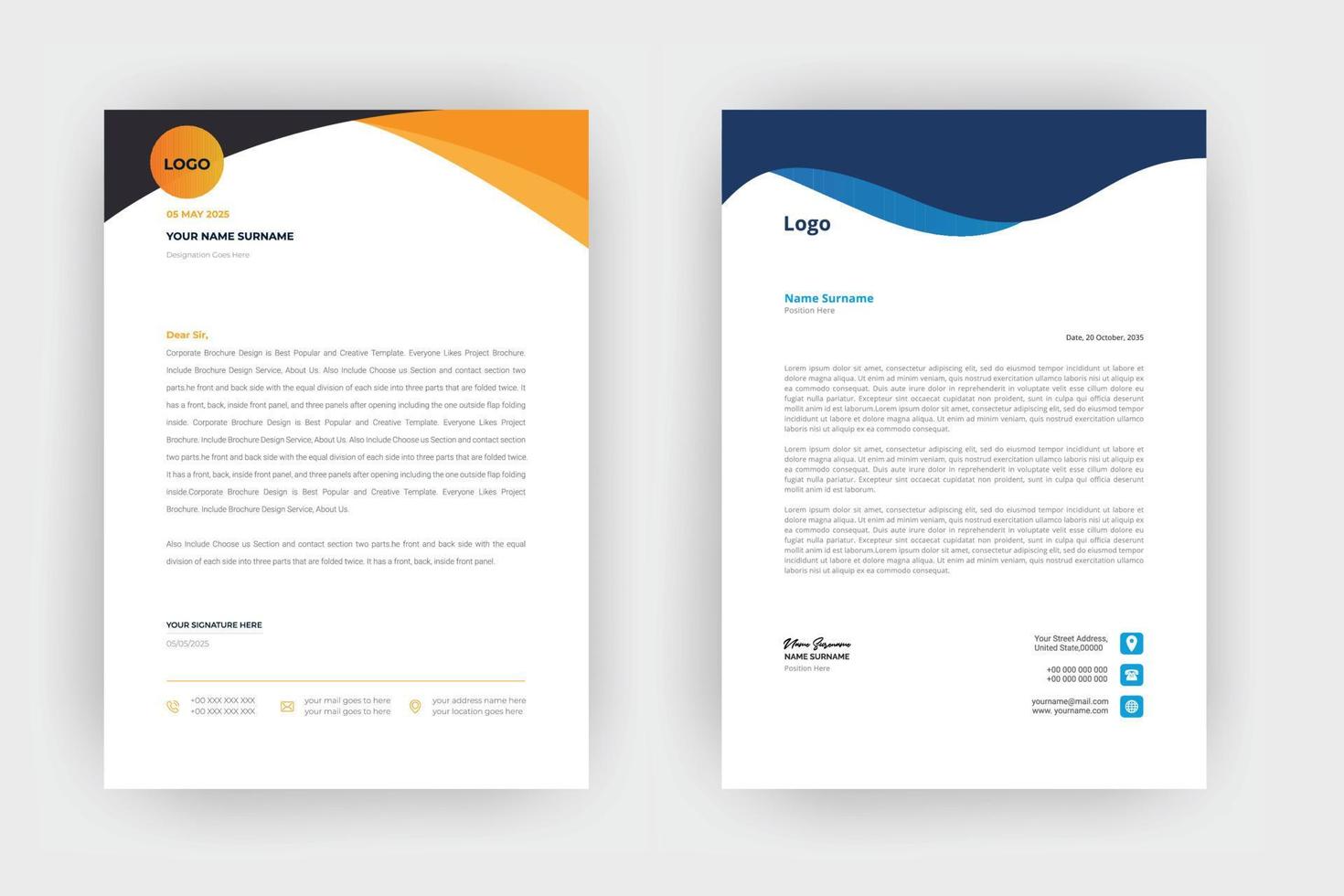The image displays two side-by-side templates for letters, positioned against a light gray background. Both templates are printed on white paper. The template on the left features a black and gold decorative header with a gold circle at the top left, containing the text "LOGO". Below the header, in dark ink, it reads "YOUR NAME SURNAME", followed by "DEAR [Recipient]". The document proceeds with a lengthy paragraph in black text and concludes with "YOUR SIGNATURE here". The template also includes accents suggesting corporate brochure design with noted colors of black, gold, and possibly blue.

The right-side template has a wavy blue pattern at the top. Beneath this, on the left, the word "LOGO" is printed in dark blue, followed by "NAME SURNAME" and a date, presumably "05, May, 2025". This template contains three paragraphs of black text and areas designated for a signature. At the bottom, there are three logos likely representing social media networks. The colors on this template range from dark blue to light blue, adding to a corporate and organized appearance.

Both templates reflect professional design elements suitable for corporate communication and are set against a minimalist gray backdrop.